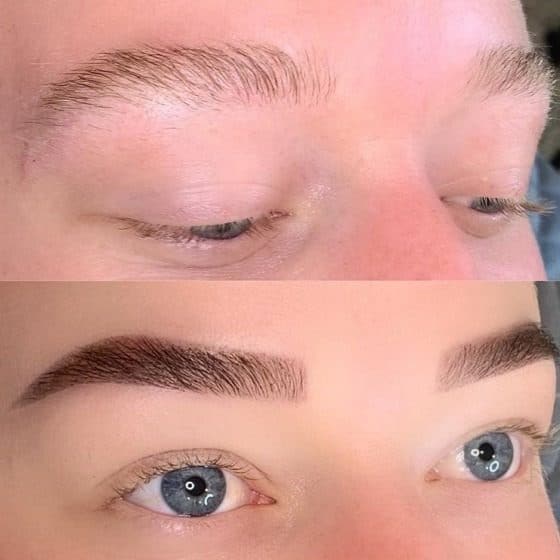The image consists of two vertically stacked close-up shots, each displaying a similar section of a person's face, from just above the eyebrows to just below the eyes. Both images focus prominently on the eyebrows and eyes of what appears to be a female with dull blue eyes. In the top picture, the person has very sparse, thin eyebrows and lashes, with no makeup on, giving a natural and somewhat unkempt appearance. Conversely, the bottom image shows the same individual, but with impeccably manicured eyebrows that have been filled in and shaped artistically, suggesting a completed beauty treatment. This transformation between the before and after shots highlights a significant improvement in the fullness and definition of the eyebrows, possibly indicating it's from an advertisement for an eyebrow salon or a eyebrow restoration service.